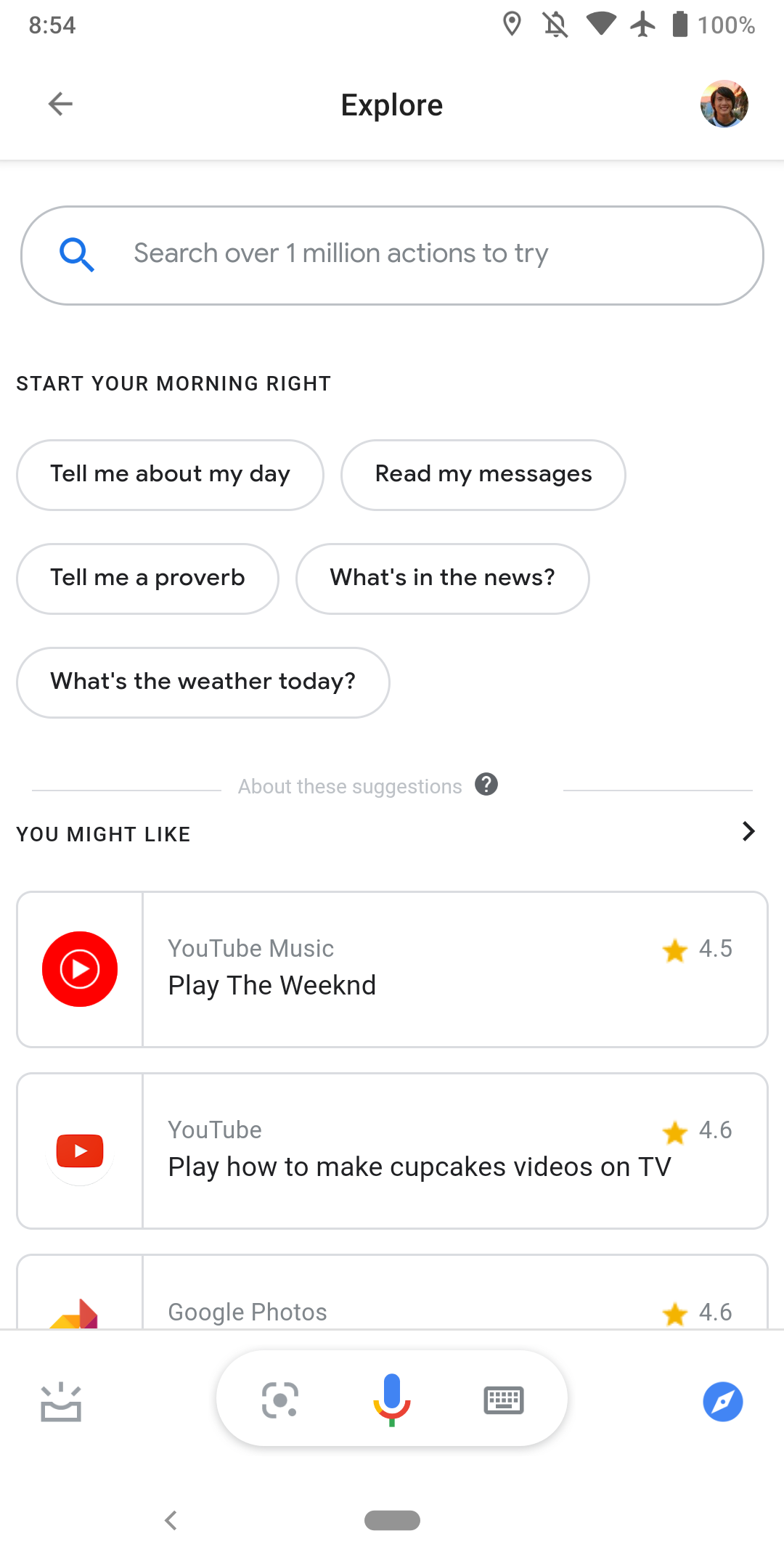A detailed photo of a cell phone screen displaying a section within the "Explore" tab. At the top of the screen is the word "Explore," followed by a search bar that invites you to "Search over 1 million actions to try." Beneath this, a section titled "Start your morning right" offers interactive options such as "Tell me about my day," "Read my messages," "Tell me a proverb," "What's in the news," and "What's the weather today."

Further down, under a heading that says "You might like," there are three suggested actions:

1. YouTube Music, identified by a red play button icon in the background and rated 4.5 stars.
2. YouTube, which suggests playing a "How to make cupcakes" video on TV, rated 4.6 stars.
3. Google Photos, partially cut off but visibly rated 4.6 stars.

At the very bottom of the screen are a microphone icon and several other icons, indicating more interactive and navigational options.